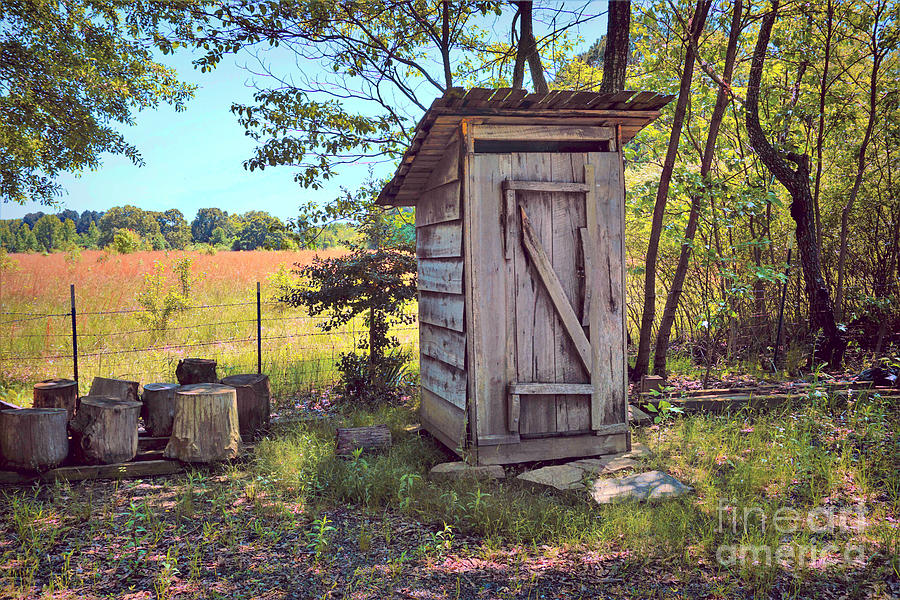The rectangular image captures a rustic outdoor farm scene dominated by an old, weathered outhouse, centrally placed against a background of natural elements. The outhouse, constructed from pale tan wood with a possibly tin or weathered wooden rooftop, lacks windows but features a single, prominent door. The structure appears tattered and worn, suggesting years of exposure to the elements.

To the left side of the frame, several tree stumps and logs are strewn about, looking like rough-hewn seating or remnants of felled trees. A small barbed wire fence runs behind the outhouse, partially enclosing a field of untamed grasses and scattered shrubs, which transition into a mix of green and orangey-brown hues. 

On the right, there is a cluster of thin trees, adding to the sense of an undisturbed environment. The scene is framed by a blue sky, enhancing the bucolic atmosphere. At the bottom right corner of the image, semi-legible white text reads "Fine Art America," subtly marking the photograph's origin.